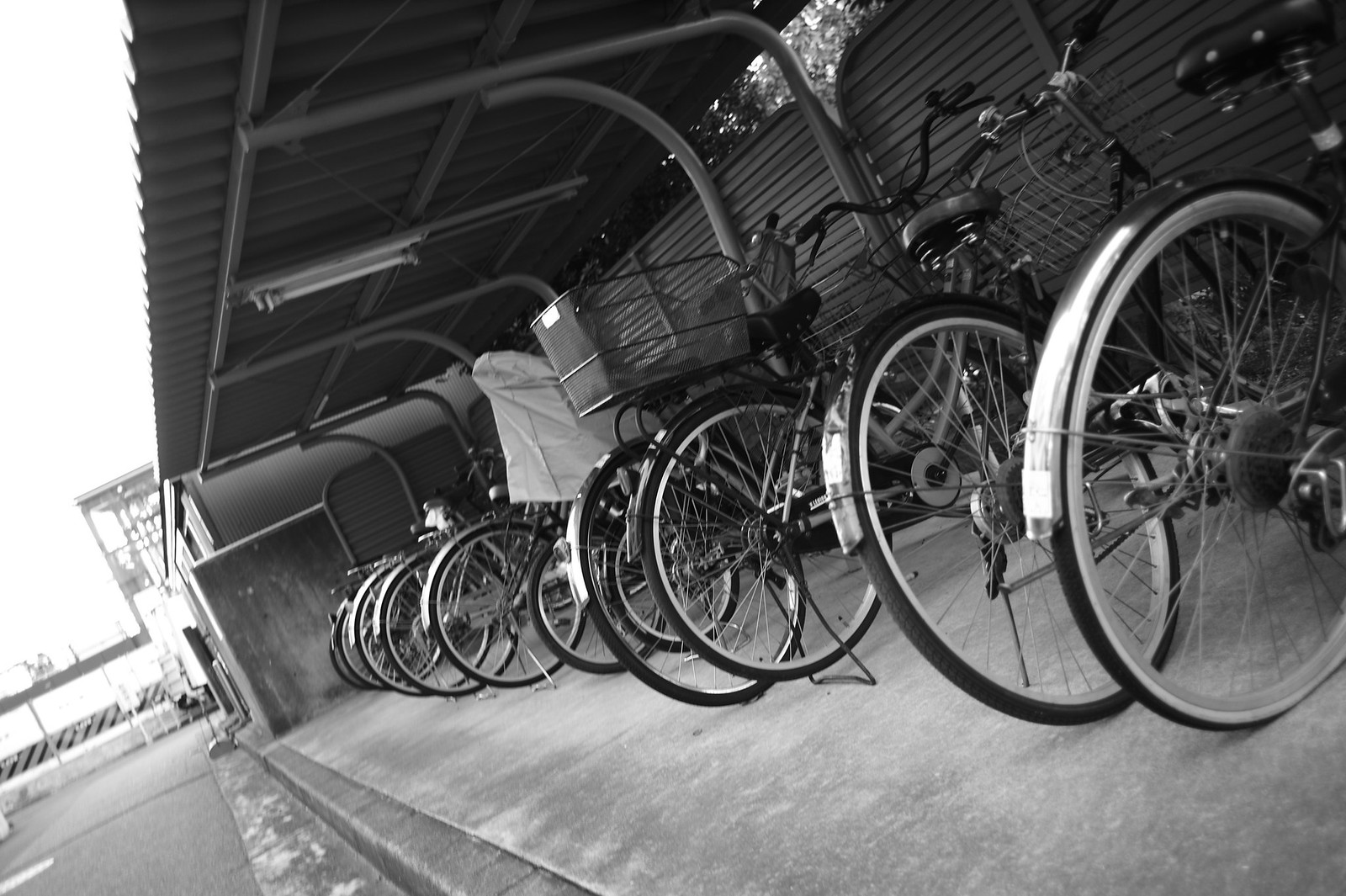The black-and-white image features a row of bicycles, approximately 10 to 12 in number, meticulously lined up on a concrete platform. These vintage-style bikes, characterized by long wheel covers over the rear tires, are parked under a protective shed that shields them from the elements. Each bicycle has its kickstand engaged, ensuring they remain upright. Several bikes sport large metal baskets, either on the handlebars or mounted over the back wheel. Notably, one bicycle has its handlebars covered and another appears to have a flat tire with white-wall tires. The setting suggests a communal storage area, possibly near a train or bus station, where people park their bikes. The image is taken from a diagonal angle, adding a dynamic perspective to the otherwise orderly scene. In the upper left corner, there is a hint of a path and possibly a bridge, further indicating the location's functionality as a transit point.